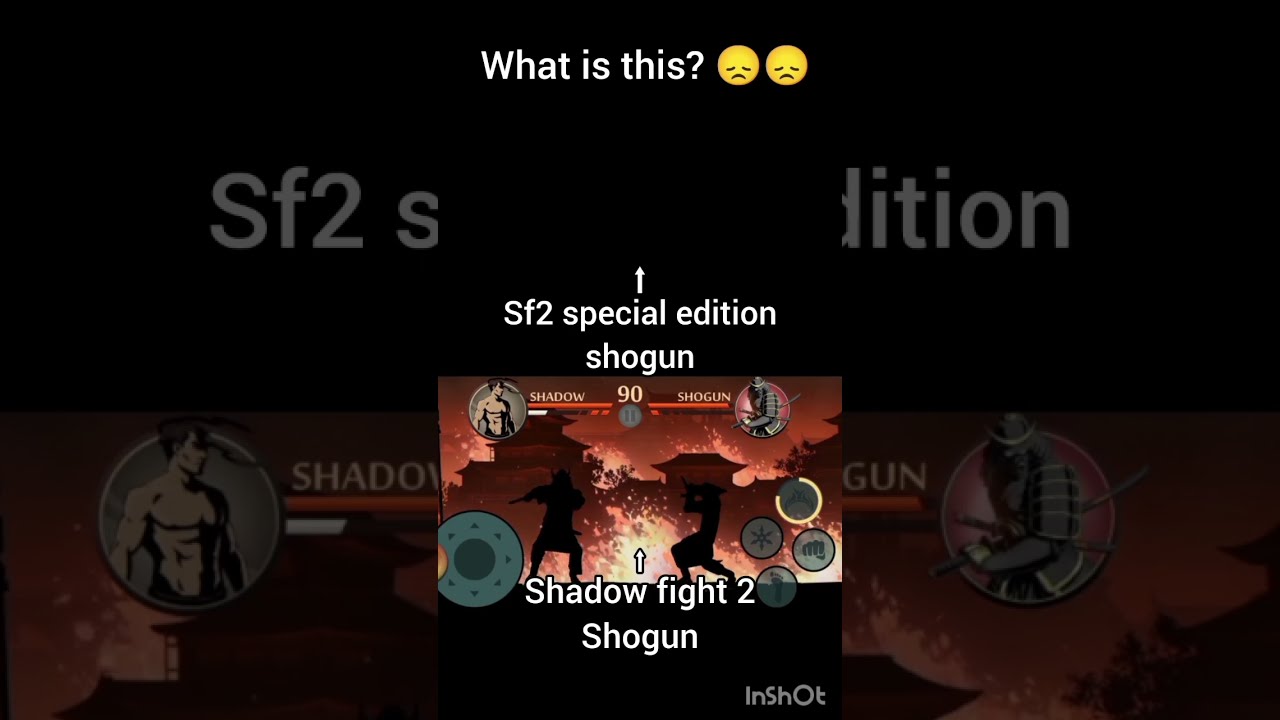The image is divided into three vertical sections, each featuring a darkened close-up of the center panel as a blurred and grayed-out border. The central section displays a screenshot from a fighter video game where two characters are battling against a backdrop of traditional Chinese or Japanese buildings. At the top of this section, white text reads "What is this?" followed by two yellow frowning face emojis. Below, the text "SF2 Special Edition Shogun" appears twice: once in off-white and once in brighter white, with overlapping text also partially visible in the side sections. Near the bottom, it says "Shadow Fight 2 Shogun," and in the bottom right corner, a watermark reads "InShot" in gray letters.